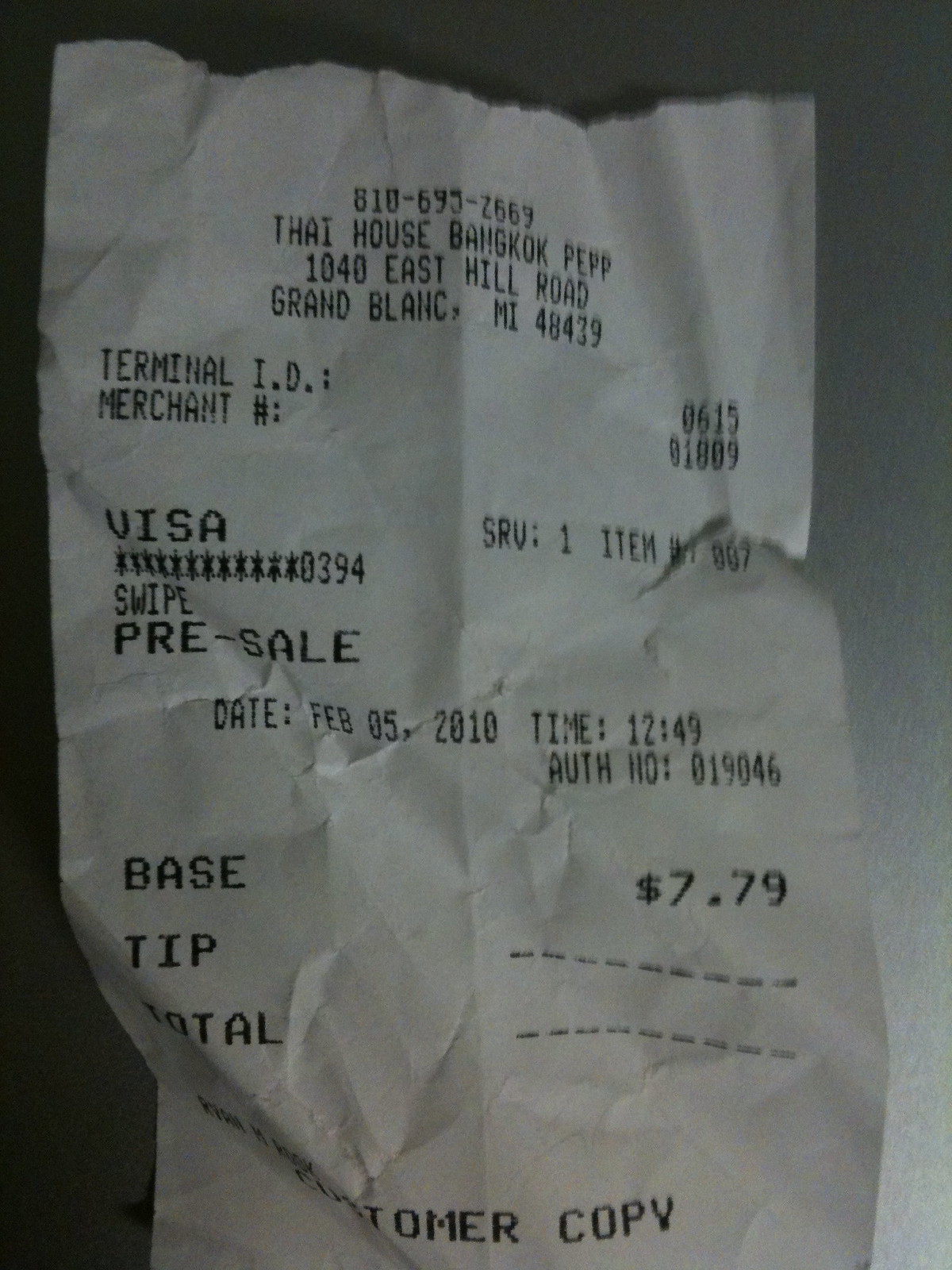This image depicts a crumpled white receipt against a gray background, primarily from a restaurant named Thai House Bangkok PEP located at 1040 East Hill Road, Grand Blanc, Michigan, 48439. At the top of the receipt, the phone number 810-695-2669 is clearly visible. Details include the terminal ID 0615 and merchant number 01809. It was a Visa card transaction with the last four digits of the card being 8394, marked as a "swipe pre-sale." The receipt also lists a server number 1 and item number 007. The transaction date is February 5th, 2010, at the time of 12:49 PM. The base price shown on the receipt is $7.79, with sections for a tip and a total amount. The receipt is identified as the customer copy.